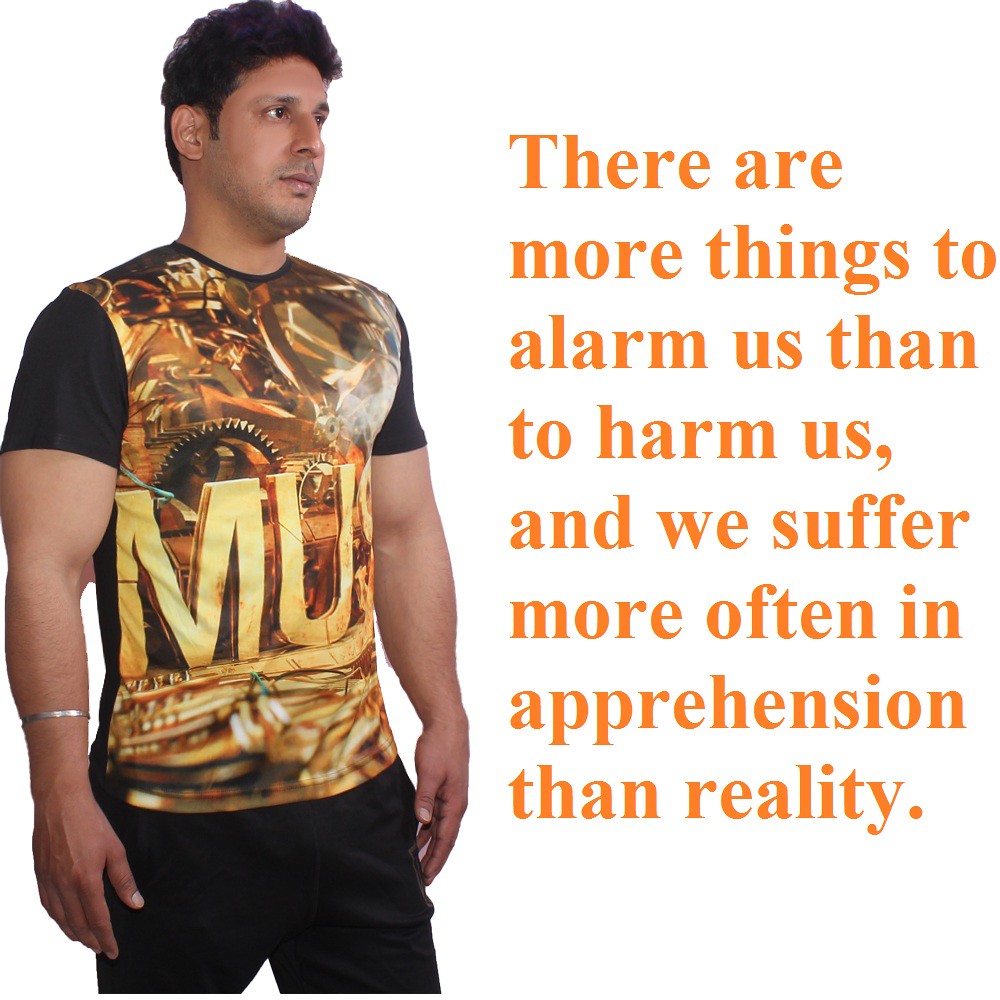The image features a man positioned on the left side and a motivational quote on the right side, all set against a white background. The man, who appears to be of Middle Eastern or possibly Indian descent, has short, curly black hair and olive-colored skin. He is muscular and faces slightly to the right, directing his gaze toward the text. He wears a multicolored shirt, primarily gold and black, adorned with images of gears and machinery parts, and the visible letters "M-U" on the front. He also sports a silver bracelet and black pants. The quote in orange text on the right reads, "There are more things to alarm us than to harm us, and we suffer more often in apprehension than reality." This striking combination of the robust figure and the thought-provoking quote creates a compelling visual contrast.